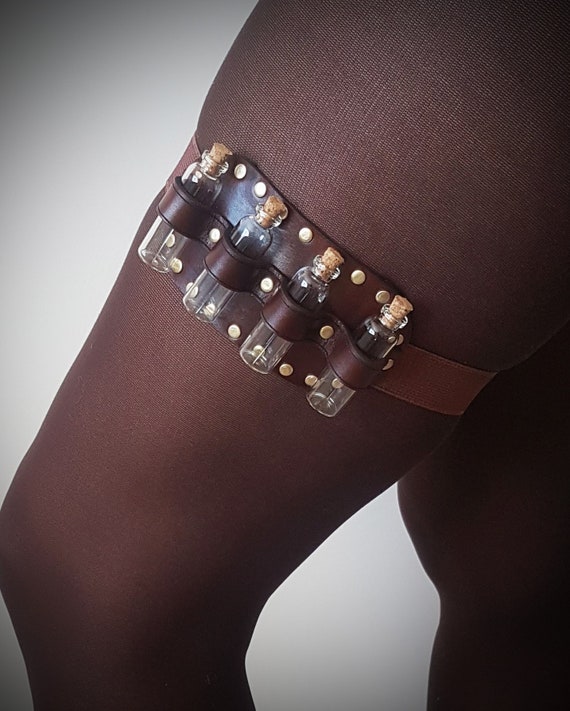This image captures the upper thigh of a person, presumably a woman, adorned in dark brown or black stockings that appear to be made of a sheer, tight fabric, given their noticeable lines and varied opacity from the kneecap up to the thigh. The focal point of the image is the thigh, where a brown leather garter belt encircles the leg. This belt is simple yet distinct, featuring a few decorative dots along its length. Four small glass bottles, each sealed with a cork, are securely fastened to the belt by thinner leather straps. The bottles are empty, resembling miniature vials possibly intended for holding substances like alcohol. The background of the image is a minimalistic, white shadowy scene, putting emphasis on the leg and the intricately adorned garter belt.